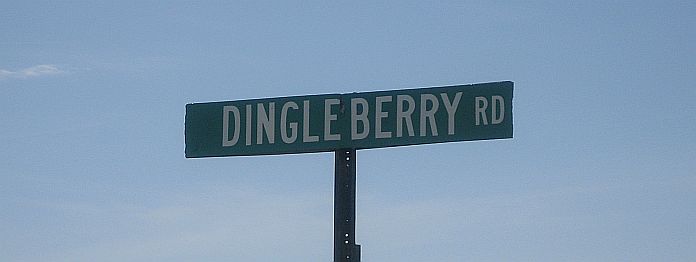The image depicts a classic American green street sign with white text that reads "Dingleberry Road." Positioned prominently against a backdrop of a light blue sky with faint hints of clouds, the sign stands out due to its simple yet recognizable design. "Dingleberry" is written in larger capital letters compared to the smaller "RD" that follows. The entire sign is mounted on a metal post, which features a series of holes and declines out of frame, suggesting it is firmly rooted in the ground. The green rectangular sign has a slender, long shape. The viewpoint appears to be slightly elevated, allowing only the top portion of the sign and part of the supporting post to be visible against the clear sky.